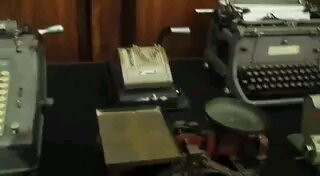The photograph depicts a museum exhibit featuring old Stynograph machines and an antiquated printer, though the image quality is blurry and out of focus, making it challenging to discern precise details. Positioned prominently in the upper right corner, there is a large, square-shaped, blocky printer with multiple detached keys on its front and a white placard facing outward. This printer has an insert for paper at the top. Adjacent to it on the left is a white, box-like machine, and further left are two more devices, one of which appears to be another typewriter with visible keys and a lever. The background showcases wooden walls with siding on the top half and possibly a black flooring at the bottom, creating a stark contrast with the metallic, silvery gray, and predominantly old-fashioned industrial aesthetic of the machines. In the center of the image, there is a cup that seems to either contain liquid or is perhaps a candle. The overall ambiance of the exhibit, although distorted by a lack of clarity and poor lighting, suggests a nostalgic look at historical office machinery.